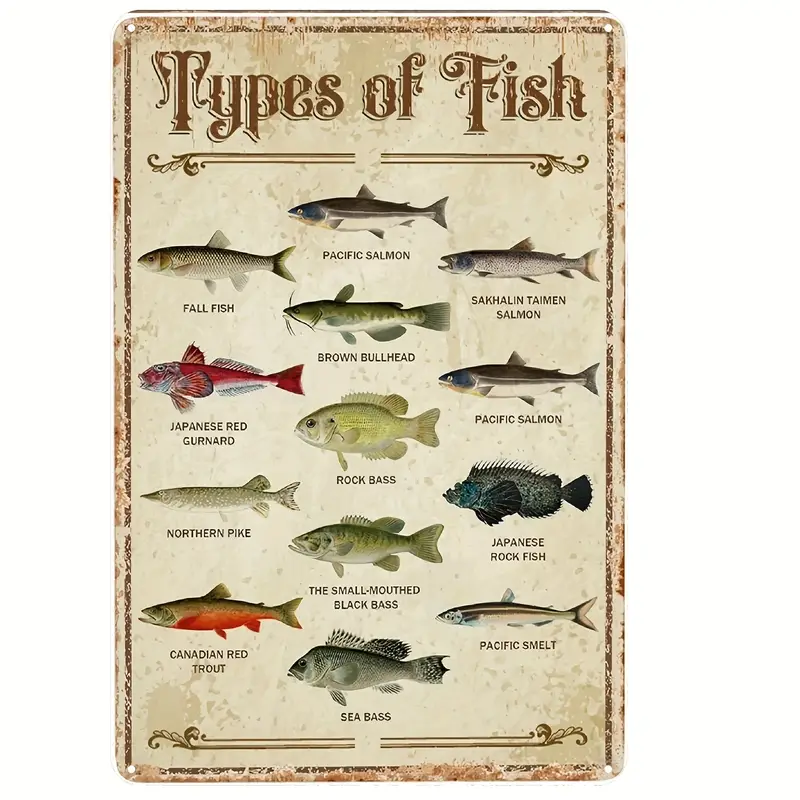This image depicts an old, rustic sign, reminiscent of vintage posters commonly found at parks or near lakes, made from what appears to be weathered metal. The sign, adorned with traces of rust, prominently features the title "Types of Fish" written in brown at the top. Below this heading, a variety of fish illustrations are meticulously detailed, each accompanied by a label identifying the species. The depicted fishes include: a blue, gray, and white Pacific Salmon, a gray Fall Fish, a distinctively shaped gray Tamien Salmon, a green and white Brown Bullhead catfish, a red and white Japanese Red Gurnard, a light green Rock Bass, a Northern Pike, a Japanese Rockfish, a Smallmouth Black Bass, a Canadian Red Trout, a Pacific Smelt, and a Sea Bass. The combination of the illustrations and the detailed names provides an informative and visually engaging overview of different fish species.